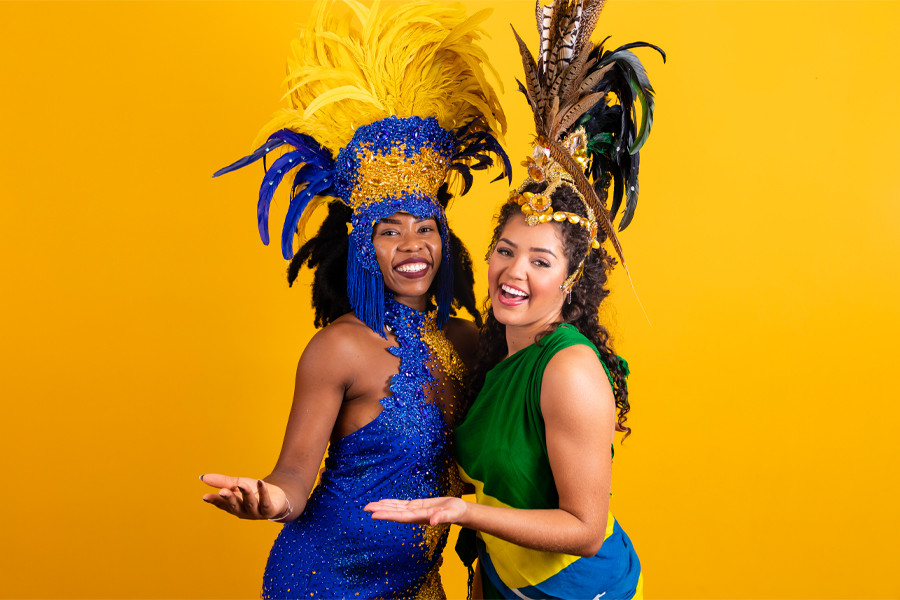The photograph features two women against a vibrant yellow-orange background, dressed in elaborate Mardi Gras-style costumes. On the left, a Black woman with shoulder-length, nappy black hair, and purple lipstick is smiling warmly. She wears a striking headdress adorned with dark blue and yellow feathers that extend about one to two feet above her head, and a matching blue and yellow dress. Her right arm extends towards the camera.

On the right, a woman with an olive complexion and long hair flowing down her back is also smiling. She dons a green, yellow, and blue dress complemented by a headdress decorated with brown, yellow, and green feathers. Her left arm is outstretched, and she appears to embrace the moment joyfully. Both women are sporting red lips, and they radiate happiness, capturing the festive spirit of their attire.